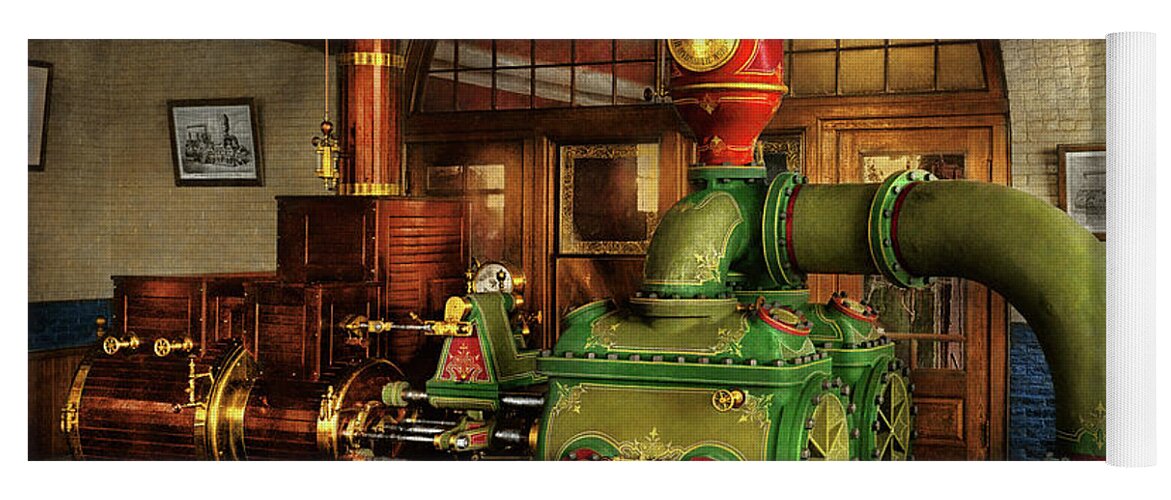The photograph showcases a large, old-timey steam engine set against a two-toned brick wall, with the left side in white and blue bricks and a picture situated on the top section. The steam engine itself dominates the image, appearing beautifully restored with intricate details. The left segment of the engine is composed of highly polished brass and copper, gleaming with a lustrous sheen. To the right, the engine features various shades of green—light green and olive green—with substantial steel tubing running throughout the structure. The top of the engine is adorned with a bright red steel train horn. In the backdrop, an old factory setting is visible, characterized by arched windows with glass panes and wooden doors beneath them. The engine also includes gold and wooden accents, further contributing to its vintage appearance. The combination of vivid colors and intricate detailing evokes a whimsical feel, reminiscent of machinery seen in fantastical settings like Charlie and the Chocolate Factory.